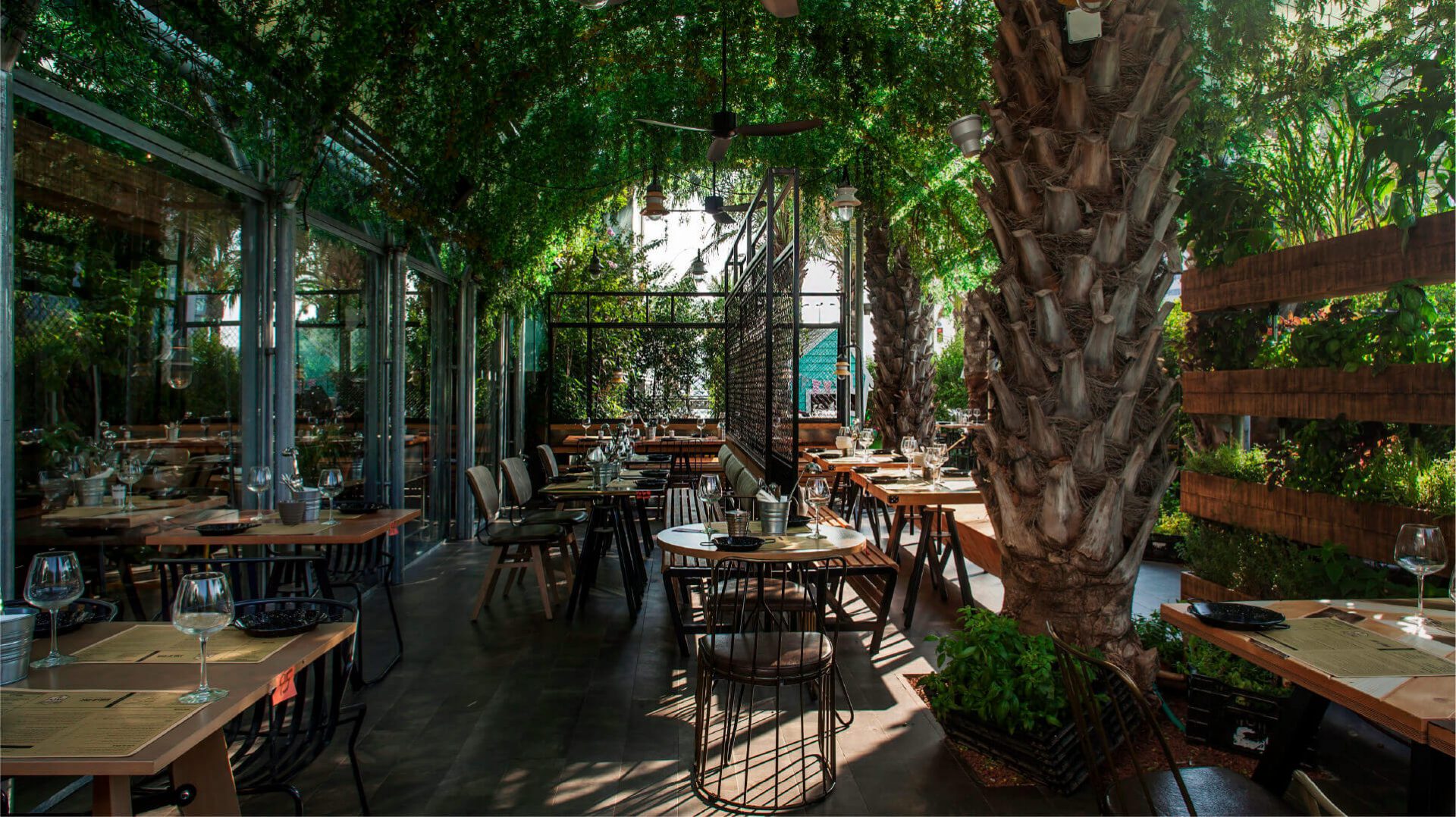The image depicts a beautifully detailed nature-themed cafe with a blend of indoor and outdoor seating areas, exuding a garden-like atmosphere. The floors are either brown or dark grayish hardwood planks, creating a warm and inviting foundation. Overhead, a canopy of lush green vines weaves across an arched ceiling, adding to the botanical ambiance. 

The seating features wooden tables adorned with clear wine glasses, metal buckets likely for silverware, and placemats or menus in beige tones. Some tables also have additional small dining accessories, possibly hinting they are being prepared for an event. The chairs have dark wood tops paired with benches and stylish brown chairs with black metal stands.

The right side of the cafe houses more seating arrangements and a prominent spiky palm tree trunk, contributing to the tropical feel. On the left, large sliding glass doors with gray frames open onto a veranda patio area filled with more green plants. This veranda, presenting an arched entry covered in vines, extends the indoor garden theme outside, seamlessly blending the natural and dining spaces. Fans with three paddles are installed on the ceiling, promoting a comfortable dining environment.

Overall, the image conveys a serene, lush, and well-prepared setting, combining elements of nature with elegant dining arrangements, perfect for a tranquil meal or a special event.